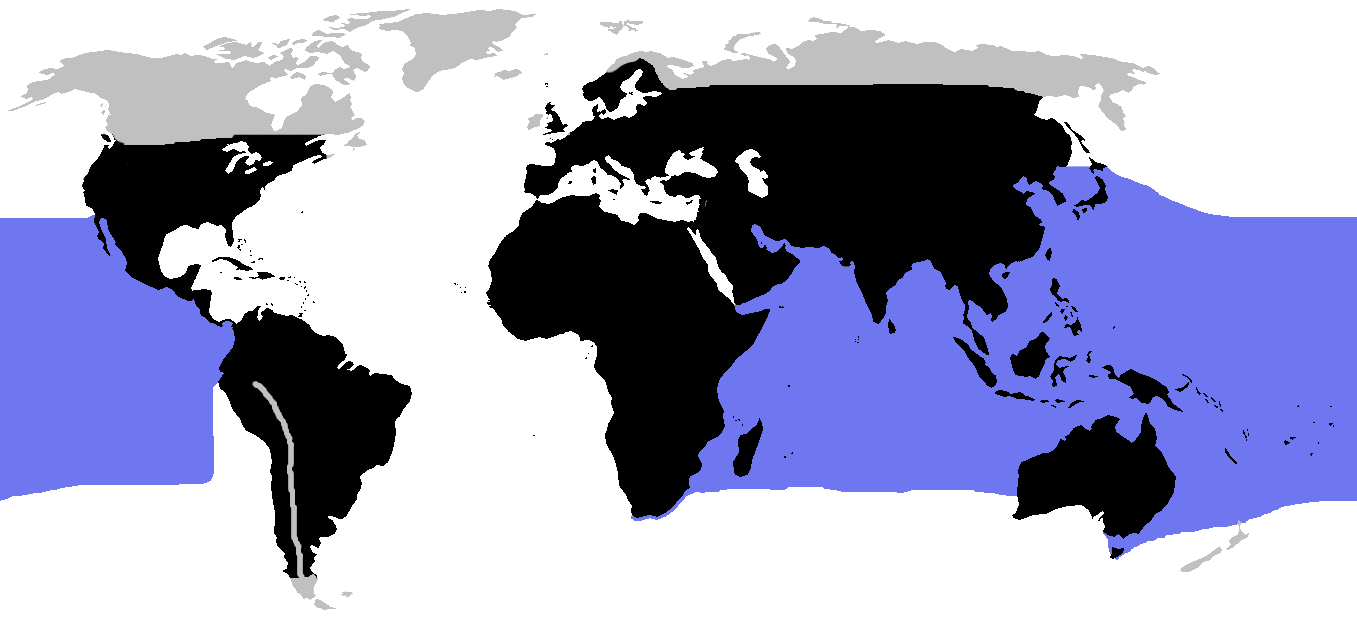This graphic features a simplified world map with a stark white background. Noteworthy color manipulations highlight various regions: Canada, Greenland, Siberia, and portions of Scandinavia are painted gray, while North America, South America, Europe, Russia, Asia, Africa, Australia, and numerous islands are rendered in black. One peculiar detail is a gray arrow drawn along the Andes mountains in Chile, pointing towards an island off the southern tip of Patagonia, also marked in gray, though its significance is unclear. Large swathes of the Pacific and Indian Oceans are shaded in blue or purple, contrasting with the plain white of the Atlantic Ocean. The map contains no labels, adding to its minimalist and somewhat enigmatic design.